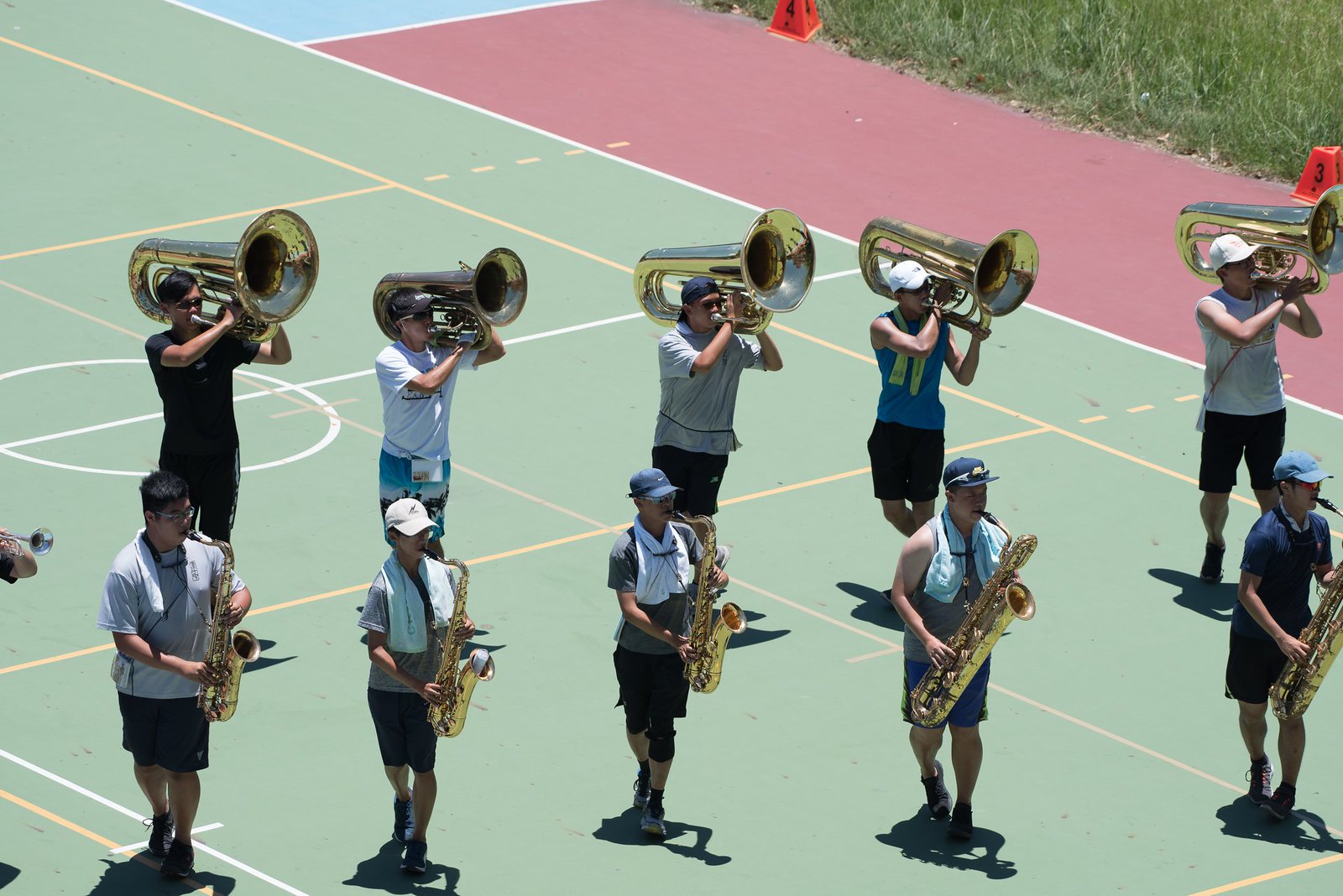This is a color photograph of a group of high school band members practicing on a green athletic court, similar but not quite like a tennis court, as there is no tennis net present. The court features a series of yellow and white lines with a prominent white circle in the middle. On the right-hand side, there's a strip of grass followed by a paved border area in blue and red, while the upper left corner has a triangle of grass with two small red cone-shaped objects.

In the image, there are ten band members arranged in two horizontal lines. The back row consists of five men playing French horns, all wearing grey or blue tops, shorts, and caps. In front of them, four individuals are playing various sizes of saxophones, dressed similarly. Most of them have towels draped around their necks to keep cool, and all but two are wearing hats. To the far left, a small part of another person can be seen. This detailed snapshot captures a moment of focused practice on the decorated court.